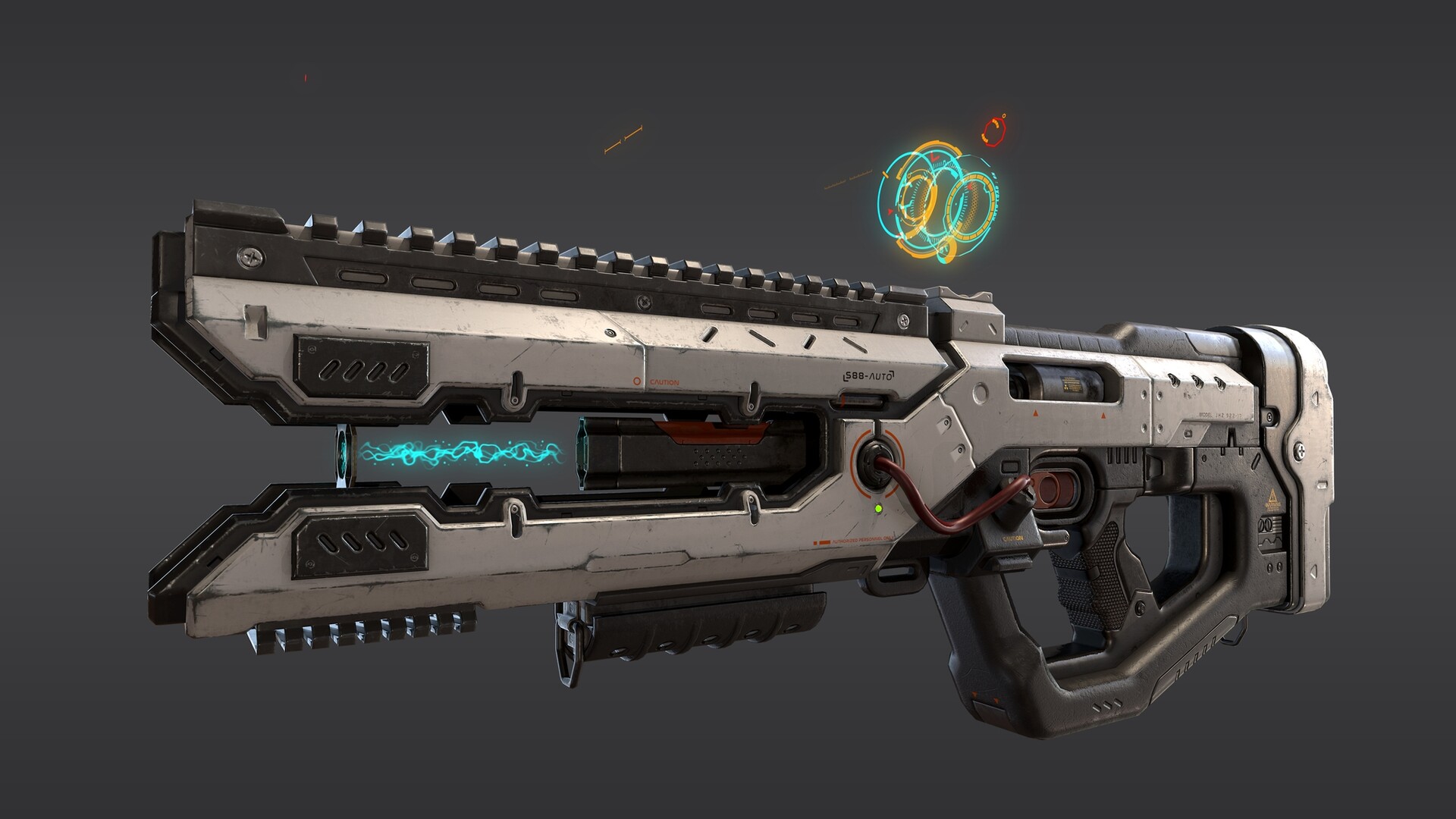The photograph showcases a futuristic, silver and black laser gun set against a dark gray background. The weapon's intricate design includes a barrel adorned with teeth-like details, reminiscent of a machine gun or a power tool. A prominent feature is the red wire extending from its left side, adding to its high-tech appearance. The gun's rear end is decorated with multicolored rings—blue, yellow, and red—emitting a sense of advanced ammunition or energy storage. Blue and yellow laser beams illuminate the front, suggesting that the gun is actively firing. There is also a noteworthy device positioned at the bottom, possibly for lighting or additional functionality. The gun has a distinct trigger, solidifying its role as a handheld weapon.